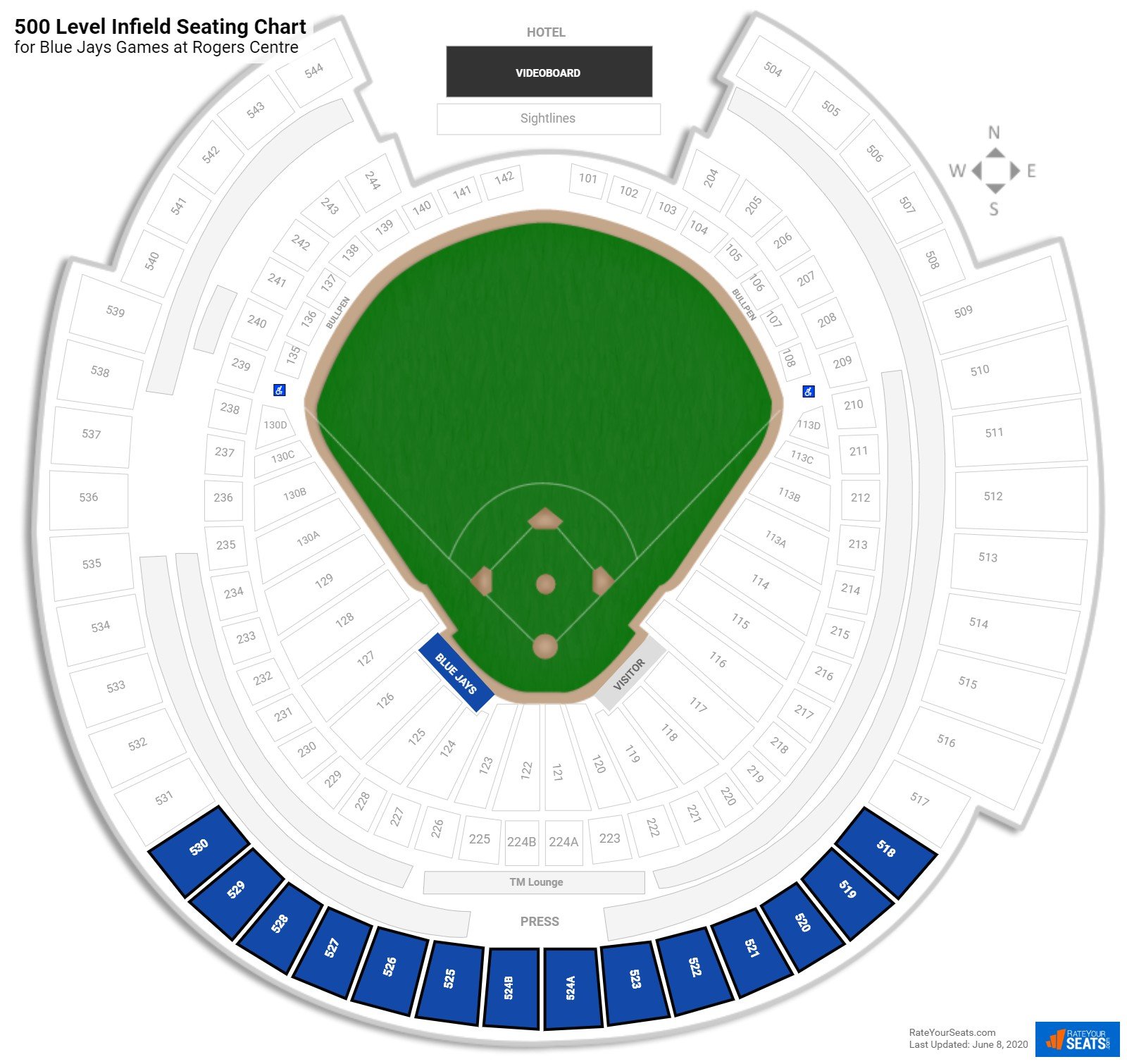The image depicts the seating view of the Blue Jays Stadium at Rogers Centre, focusing particularly on the 500 level infield seating chart for Blue Jays games. The baseball diamond is clearly visible, surrounded by various seating arrangements. Highlighted in blue are specific seats located behind home plate, positioned in the back section, commonly referred to as the "nosebleeds," which is the 500 level. The field itself is green, while the majority of the seats are white, except for the highlighted blue ones.

The seating chart illustrates an ascending order as you move closer to the field, starting from the 100 level near the field, followed by the 200 level, and so forth. Notably, there's a lounge situated behind home plate, positioned between the second tier, or the 200 levels. At the top center of the seating chart, a hotel video board is depicted. Additionally, the chart includes sight lines, which can be toggled on and off, to display what different sections can and cannot see. The Blue Jays' dugout is shown located between home plate and third base, positioned on that side of the field.